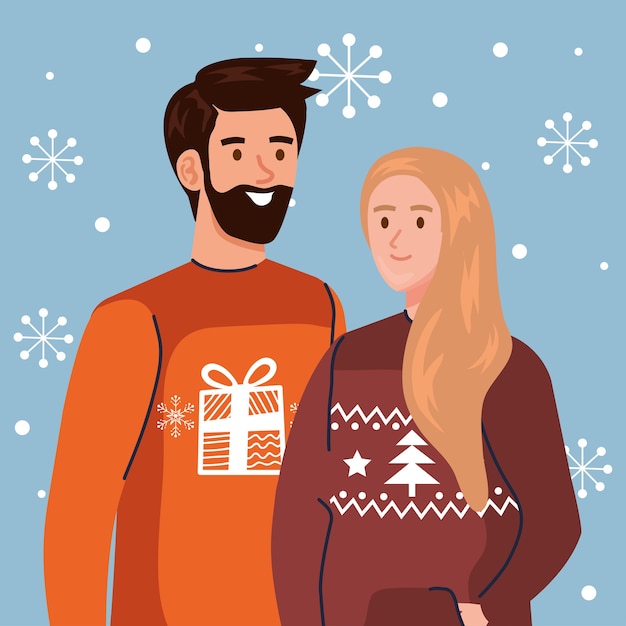This image seems to be a digitally drawn or cartoon picture of a festive Christmas scene, portraying a joyful couple standing side by side against a blue background filled with detailed white snowflakes and occasional white circles. The man, who has short brown hair and a brown beard, is depicted in an orange sweater adorned with a white present box design. He is smiling warmly while looking towards the woman beside him. The woman, depicted with blonde hair, is dressed in a maroon or dark red hoodie-type sweater with a unique Christmas design: a white Christmas tree topped with a star, surrounded by zigzag lines and small dots. She is smiling and looking directly at the man, with one hand casually placed in her sweater pocket. The image captures the festive and warm spirit of Christmas and seems well-suited as a greeting card or holiday-themed illustration.